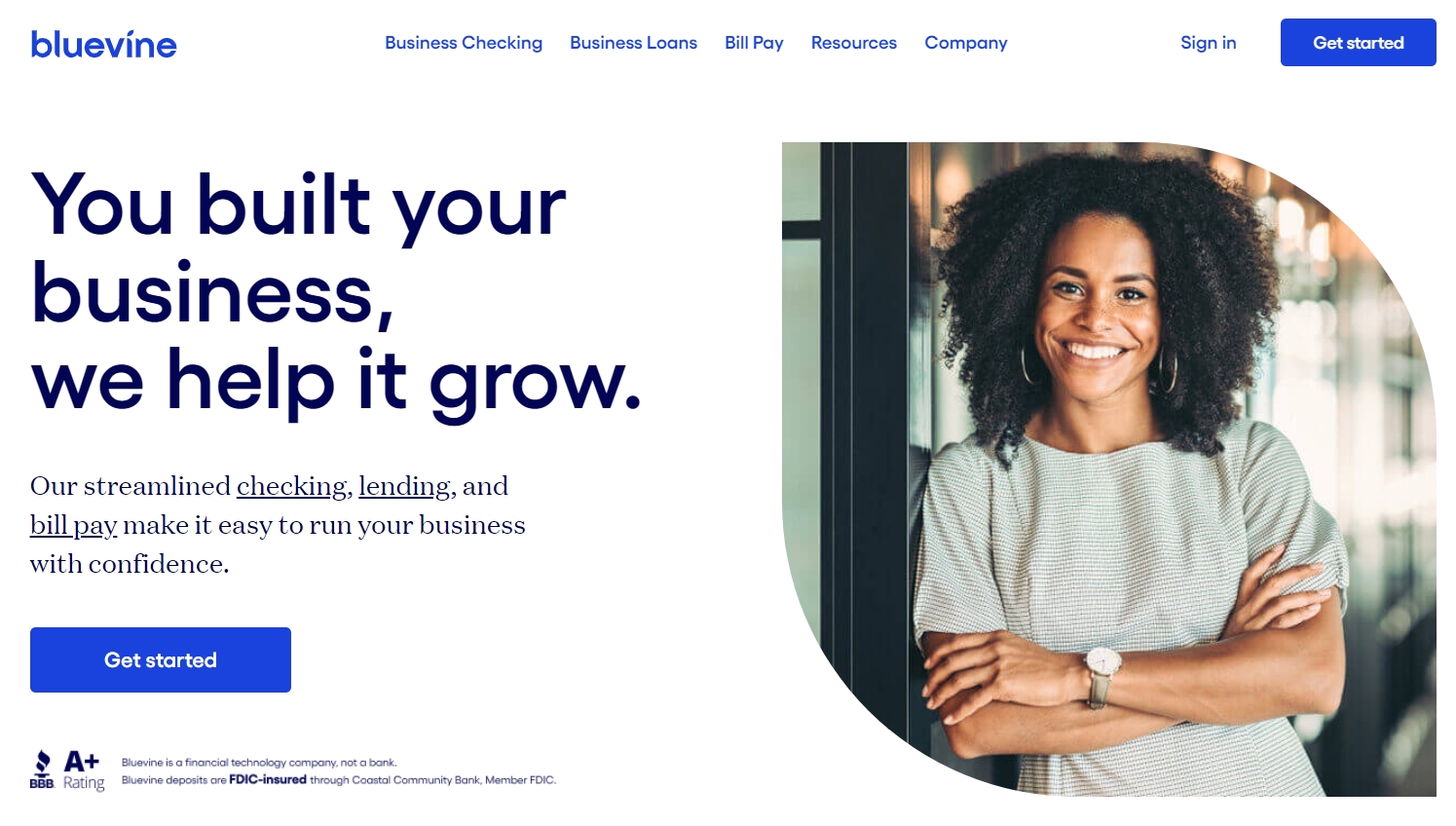The image displays the homepage of a website named "Blue Vine," with their logo prominently featured in blue in the top left corner. To the right, there is a navigation menu with options in smaller fonts, including "Business Check-In," "Business Loans," and "Bill Pay Resource and Company." Further to the right are the "Sign In" and "Get Started" buttons, the latter of which is white text on a blue button.

Below this header, a smiling black woman with folded arms leans casually against a wall. She is wearing a wristwatch and a white, striped shirt, and accessorizes with dangling earrings.

To the left of the woman, in large, bold font, are the words broken into three lines: "You built your," "business," and "we help it grow." Below this, in smaller text, it states: "Our streamlined checking, lending, and bill pay make it easy to run your business with confidence." Directly beneath this is another "Get Started" button.

Additionally, there is a Better Business Bureau A+ rating displayed, and a disclaimer that Blue Vine is a financial technology company, not a bank, with deposits being FDIC insured through Coastal Community Bank.

The overall background is white, and key elements like the Blue Vine logo and various "Get Started" buttons stand out in blue. The larger "Get Started" button appears more prominently compared to the one in the top right corner.